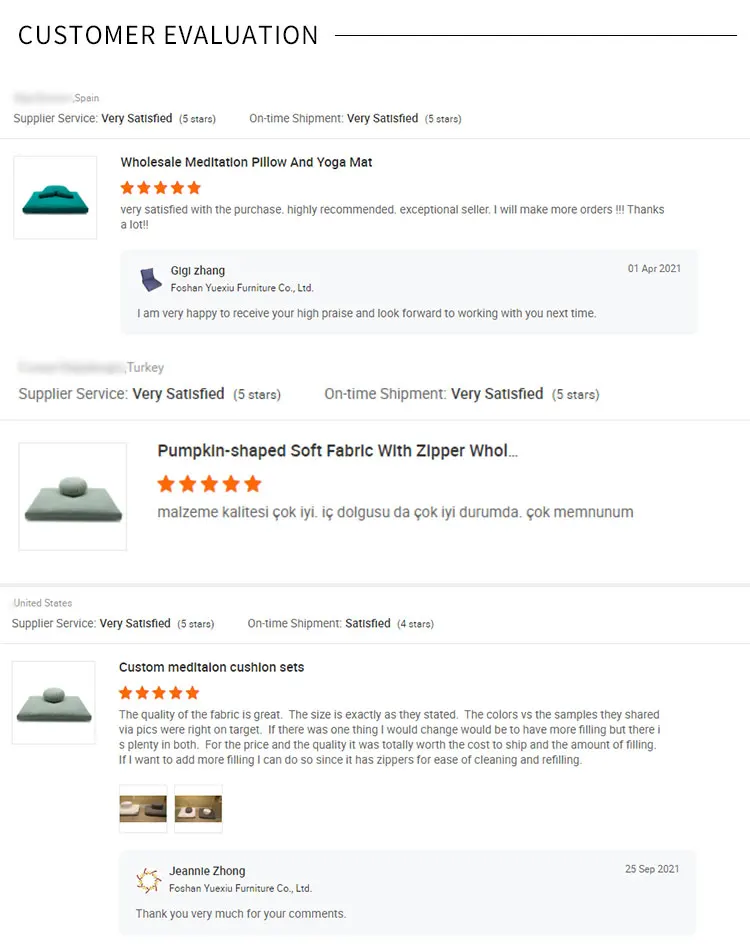**Detailed Customer Reviews for Meditation Products**

**Screenshot Overview:**

At the top of the screenshot, captured from a desktop, laptop, smartphone, or tablet, the header reads "Customer Evaluation" in bold black text, underlined by a black line. Below, part of the content is blurred and faded, indicating this review is from Spain.

**Customer Review from Spain:**

- **Supplier Service:** Very interested (★★★★★)
- **On-Time Shipment:** Very satisfied (★★★★★)

An image beside the review showcases a green meditation pillow and yoga mat.

**Product Details:**

- **Product Name:** Wholesale Meditation Pillow and Yoga Mat
- **Rating:** ★★★★★

**Customer Feedback:**

"Very very satisfied with the purchase. Highly recommended, exceptional seller. I will make more orders!!! Thanks a lot!!"

**Seller Response:**

Profile picture of a bluish yoga mat

- **Responder:** Gigi Zhang from Foshan Yuexiu Furniture Co. LTD
- **Response:** "I'm very happy to receive your high praise and look forward to working with you next time."

**Customer Review from Turkey:**

- **Supplier Service:** Very satisfied (★★★★★)
- **On-Time Shipment:** Very satisfied (★★★★★)

An image beside the review depicts a dark gray yoga mat with a darker gray border.

**Product Details:**

- **Product Name:** Pumpkin-shaped Shop Fabric with Zipper
- **Rating:** ★★★★★

Comment in Turkish provided, content not translated.

**Customer Review from United States:**

- **Supplier Service:** Very satisfied (★★★★★)
- **On-Time Shipment:** Satisfied (★★★★)

An image beside the review showcases two meditation cushions, one white and one gray.

**Product Details:**

- **Product Name:** Custom Meditation Cushion Sets in Dark Gray
- **Rating:** ★★★★★

**Customer Feedback:**

"The quality of the fabric is great. The size is exactly as stated. The colors versus the samples they shared in pictures are right on target. If there was one thing I would change, it would be to have more filling, but there is plenty in both for the price and the quality was totally worth the cost to ship. If I want to add more filling, I can do so since it has zippers for the case, cleaning, and refilling."

**Seller Response:**

Profile picture has a sun symbol next to the name

- **Responder:** Jeannie Zhong
- **Response:** "Thank you very much for your comments."
- **Date of Response:** 25th September 2021